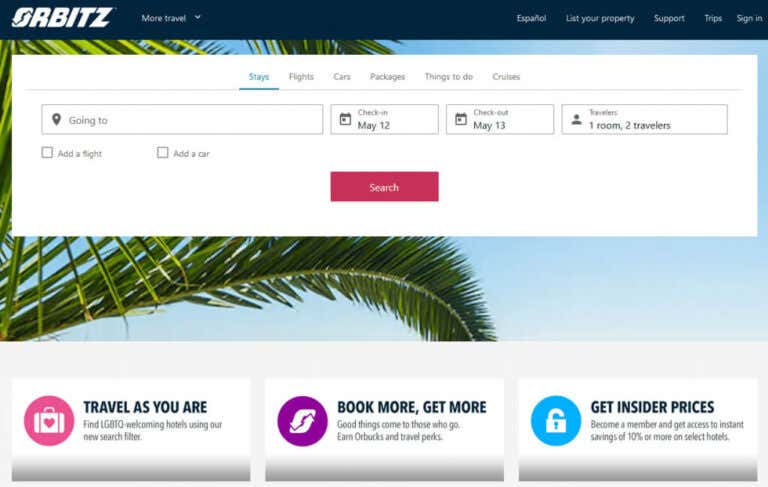This is a screen capture of the Orbitz website, a travel booking platform. The top navigation menu includes options such as "List Your Property," "Support," "Trips," and "Sign In." Users can choose to view the website in Spanish. The search bar provides categories for "Stays," "Flights," "Cars," "Packages," "Things to Do," and an additional unidentified option starting with the letter "C." The main display features an image of a clear sky and palm fronds. Below the image are input fields for booking details: the destination, departure date of May 12th, return date of May 13th, one room, and two travelers. The search button is prominently displayed. Further down, there are additional promotional links with phrases such as "Travel As You Are," "Book More, Get More," and "Get Insider Prices."